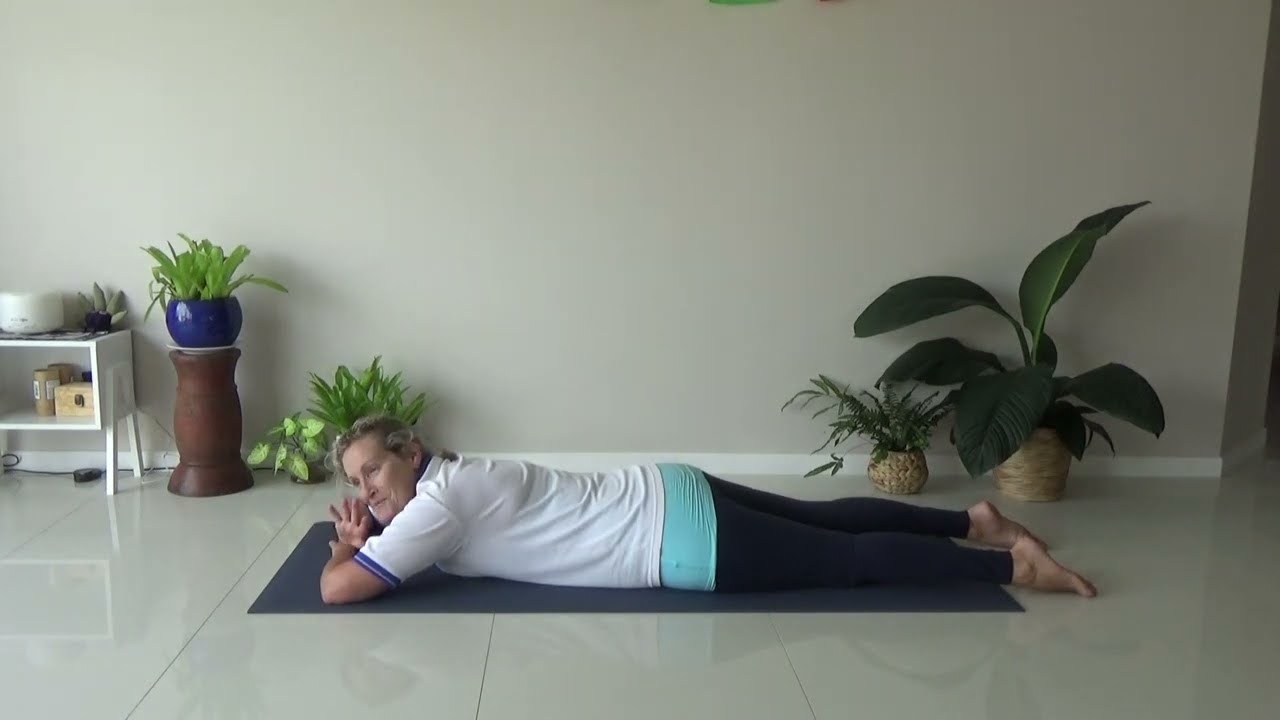In a serene indoor setting, this image captures a woman practicing yoga on a sleek, shiny white tile floor, reflecting the various elements around it. The back wall, a light beige or tan color with white molding at the base, serves as the backdrop. To the left, a small bookcase houses undefined objects and succulents, while beside it, a wooden pedestal displays a navy blue pot with vibrant green plants. On the right, wicker baskets hold lush plants with large green leaves.

Centered in the composition, the woman lies on a thin black yoga mat, her body stretched out with her legs extended behind her. Resting on her elbows, she turns her head slightly towards the camera, showcasing her light blonde hair and a gentle, subtle smile. She wears a white short-sleeved shirt edged in dark blue and black leggings with a mint green band at the top. Her relaxed pose and the tranquil environment suggest a peaceful moment of self-care and mindfulness.